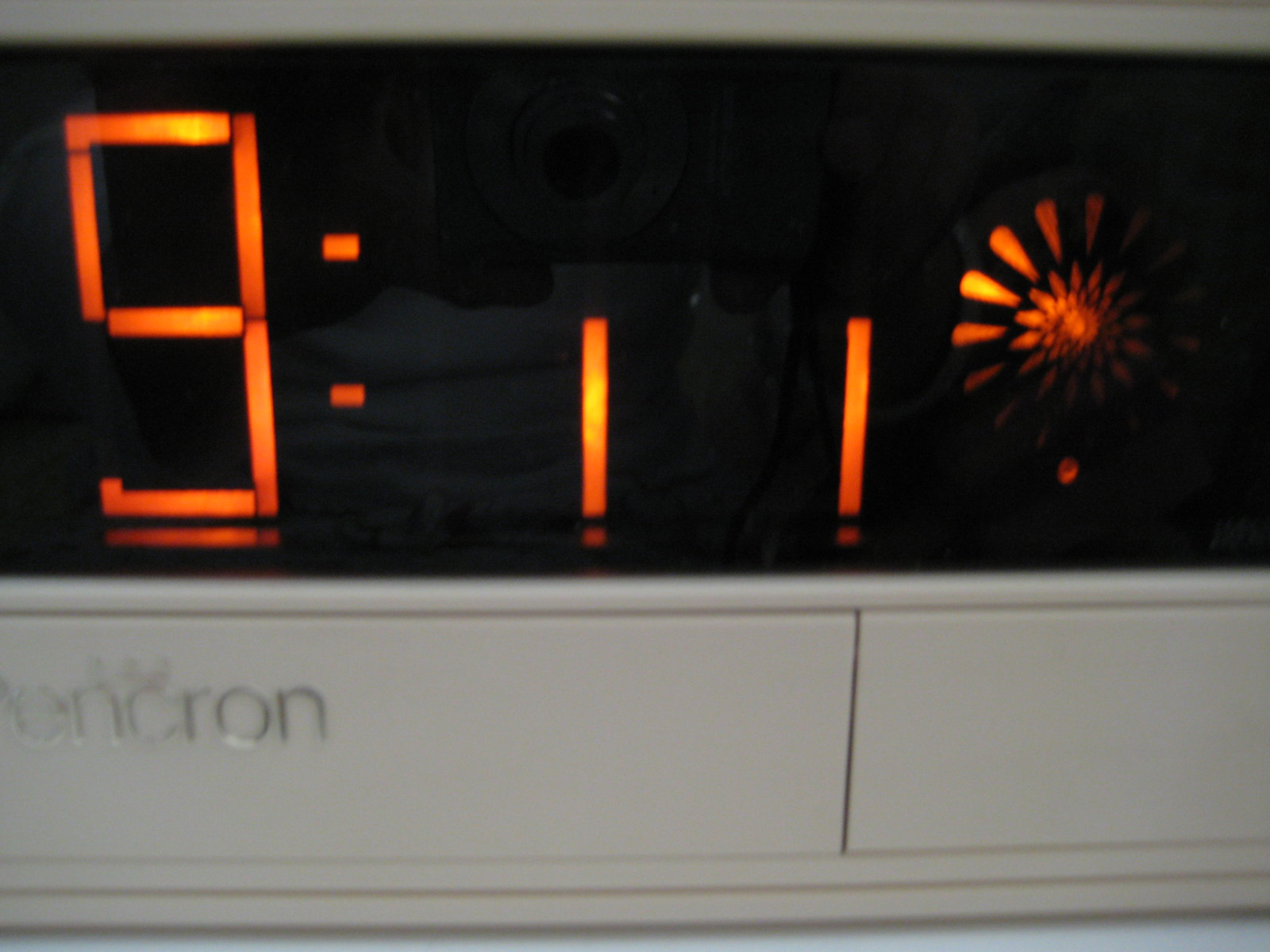The image depicts a close-up digital clock or alarm against a predominantly black background. The time is displayed in orange, with a prominent "9" followed by two dots (colon), and then two "1"s with partly faded tops, indicating possible light malfunction. Adjacent to the time display, there is a circular starburst shape resembling a sun or fireworks in the same orange hue, with hints of yellow, suggesting a decorative element. The device's display screen is encased in a sleek white frame, contrasting sharply with the dark background. Below this digital screen, in the bottom left corner, the brand name "ENCRON" is etched in silver letters, though partially obscured, with the letter "C" featuring an accent mark on top. The overall design implies a primarily silver electronic device, with further sections and dividers visible beyond the main clock interface.